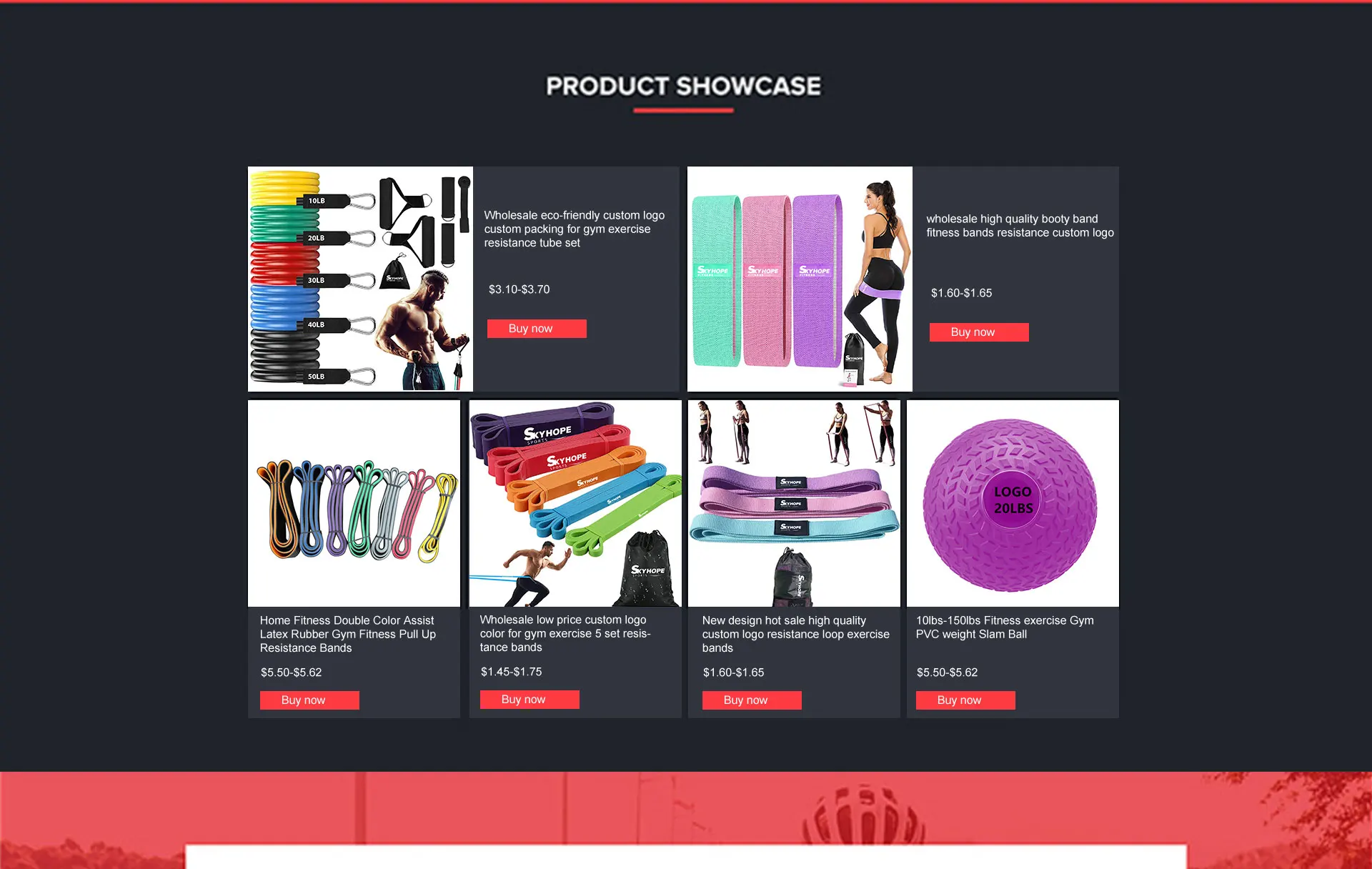This screenshot features a promotional page for various types of exercise equipment, with a visually appealing design and detailed product descriptions:

At the top, the page has a sleek black background with the text "Product Showcase" in bold white letters, underlined by a striking red line. 

In the top left corner, there is a photo collage displaying different weights, straps, and other gym equipment. It also features a shirtless man in gym shorts demonstrating the use of the equipment. The accompanying text reads, "Wholesale Eco-Friendly Custom Logo Custom Packing for Gym Exercise Resistance Tube Set," and lists the price range from $3.10 to $3.70. A prominent "Buy Now" button is located beside this description.

To the right, another image shows resistance bands in various colors: light blue, pink, and purple. A woman dressed in athletic clothing is standing near the bands. The text beside her reads, "Wholesale High-Quality Booty Band Fitness Bands Resistance Custom Logo," along with pricing information and another "Buy Now" button.

The bottom section of the page displays three more images side-by-side, with a fourth one adjacent to the row:
1. The first image features seven different colors of resistance bands.
2. The middle image showcases five different colors of resistance bands, below which is a photo of a shirtless man in sweatpants using one of the bands.
3. The third image contains more resistance bands, along with photos of people using them.
4. The final image in the row depicts a purple slam ball with the label "Logo 20 Pounds."

Each product is clearly highlighted with specific details, enticing visuals, and call-to-action buttons, designed to attract potential buyers.